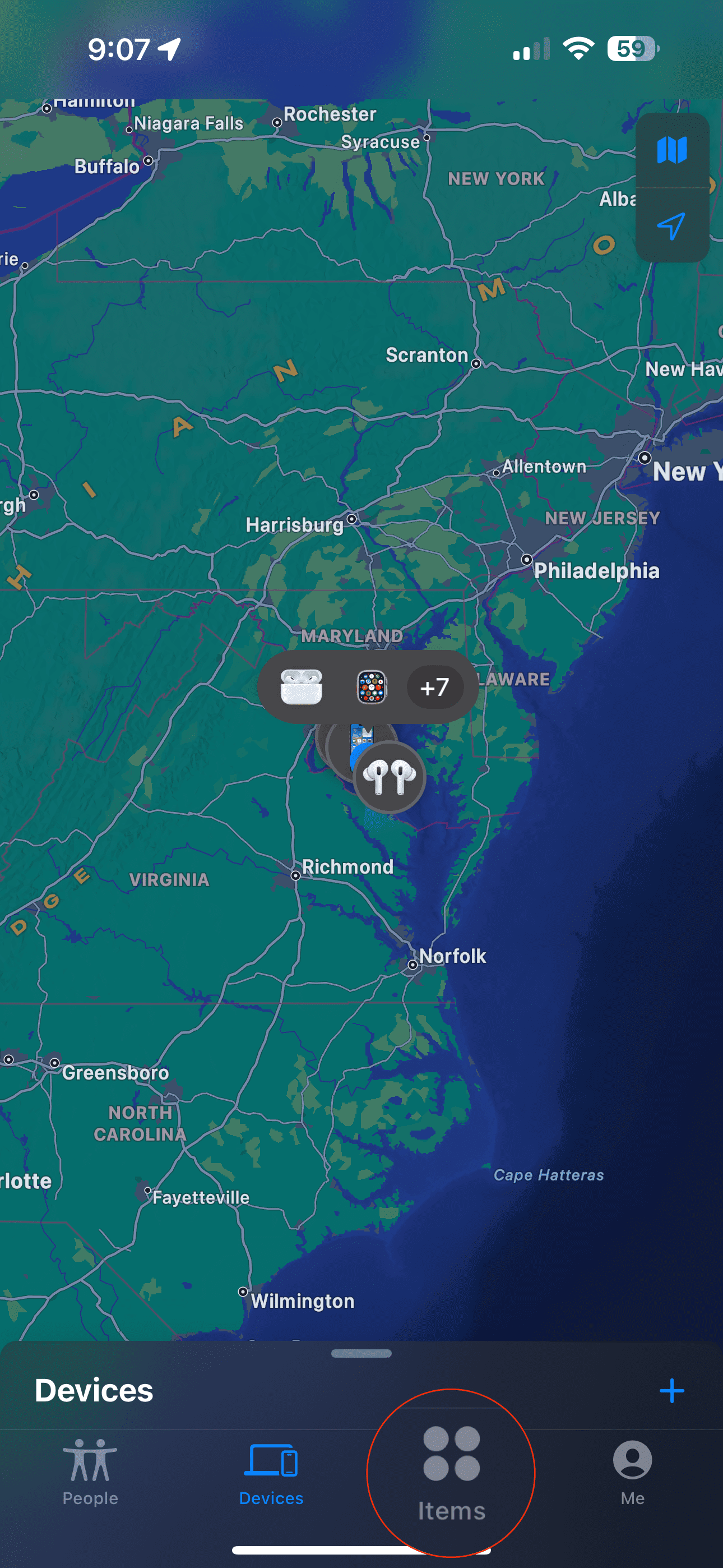This screenshot features a detailed map predominantly colored in shades of dark midnight blue and varied greens. The map highlights a body of water located in the lower right corner, while the land spanning from the south includes notable locations such as Wilmington, Cape Hatteras, Norfolk, Richmond, Delaware, Virginia, Maryland, Philadelphia, Harrisburg, New Jersey, Allentown, New York, Scranton, Albany, Syracuse, Rochester, and Buffalo, extending up to Niagara Falls in the upper left corner. At the bottom of the screen, there are icons labeled "People," "Devices," "Items," and "Me," indicating the different categories that can be accessed.